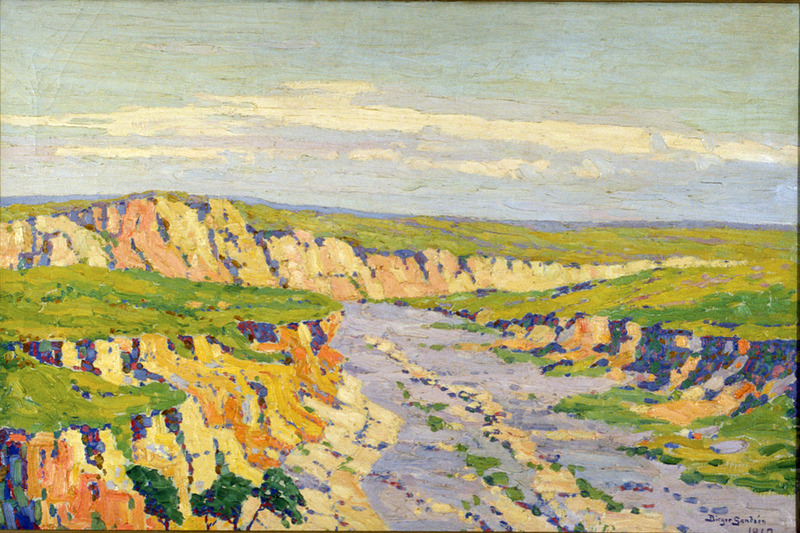This image is a whimsical painting saturated with vibrant colors, depicting a semi-abstract natural landscape. In the background, a sky filled with light baby blue tones is adorned with wispy white clouds. Dominating the scene are three distinct rocky mountains, with sections covered in green grass indicating a natural terrain. These digital-looking clip art mountains, though not realistic, exhibit earthy brown hues and signs of erosion along their sides. Nestled between two of the mountains is a meandering, shallow river, characterized by patches of green vegetation on rocky outcrops within the water, suggesting low water levels. Towards the bottom-left corner of the picture, a few small trees and bushes add detail to the earthy foreground. Beyond the rocky mounds and hills, a darker navy blue stretch hints at a distant ocean, creating depth in the composition. Signed at the bottom right, the artist's name appears, albeit faintly, as "Beery Sundown."